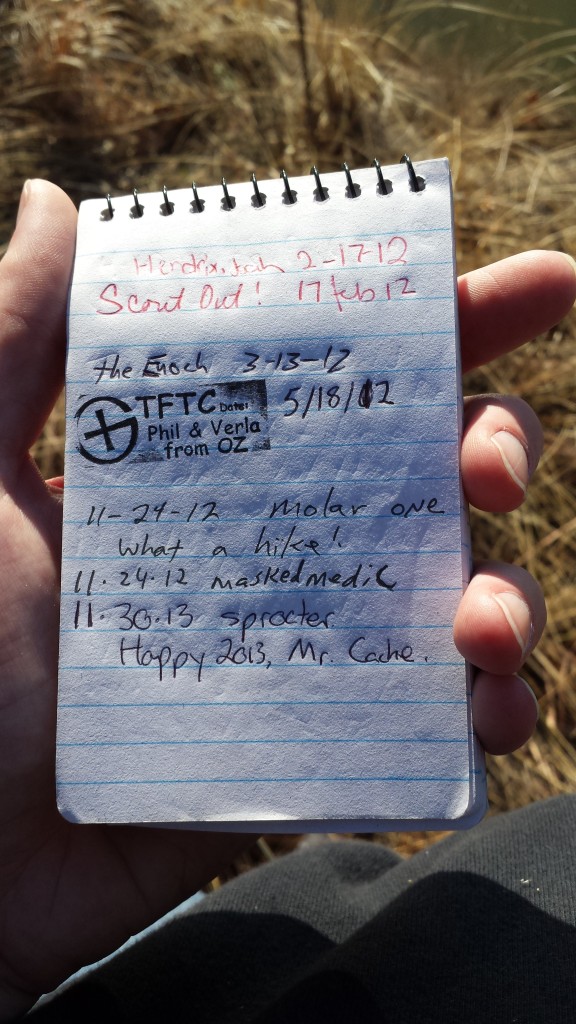The image is a close-up, vertical shot of a person's hand holding a small spiral-bound notebook with lined paper. The notebook, small enough to fit in a shirt pocket, has handwritten notes in both red and black ink. At the top of the first page, there are several dates and events listed, though the handwriting is somewhat difficult to decipher. The background reveals an outdoor setting, likely a trail or overgrown field strewn with brown stones and weeds. The hand, centrally positioned in the frame, shows the thumb and three fingers gripping either side of the notebook. The image captures soft earthy tones, including browns from the setting and hints of colors from the person's outfit, suggesting a daytime scenario.